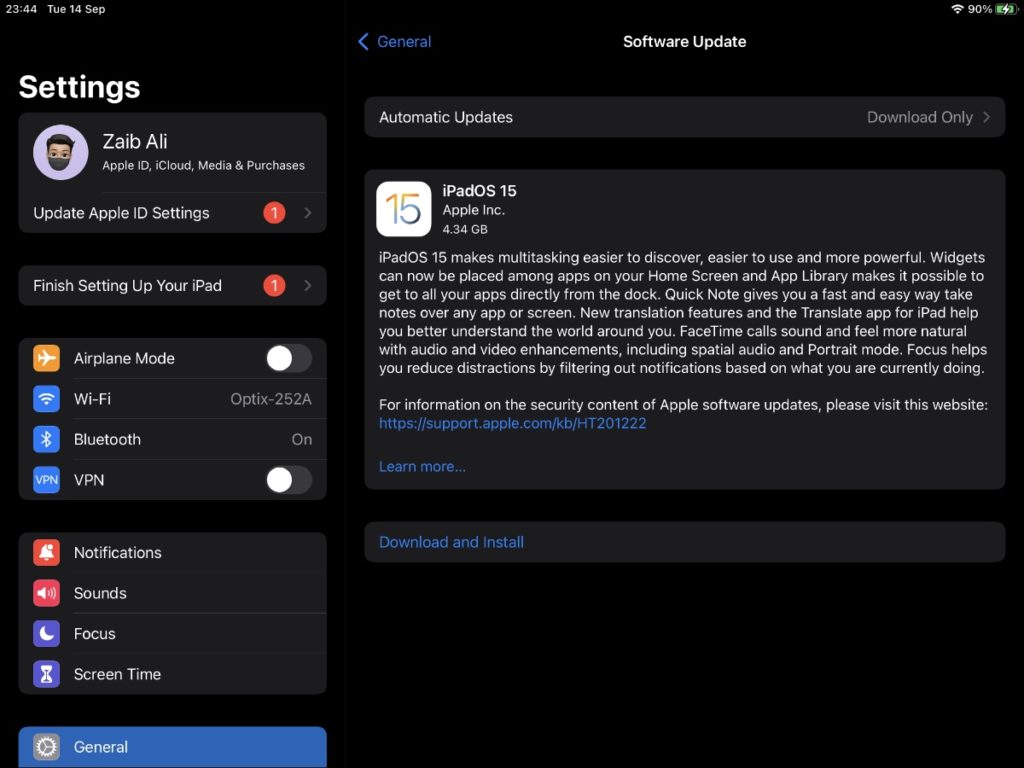This image shows a detailed view of the settings page from someone's iPad. At the top, the profile section features a circular avatar with the name "Zayab Ali." The avatar depicts a person with darker skin, black hair, and black eyes, who is wearing a health mask over their face. Just below the profile picture, various options are visible, including "Apple ID," "iCloud," and "Media & Purchases." There is a notification in a red circle indicating a need to "Update Apple ID Settings" and another notification to "Finish Setting Up Your iPad."

Moving further down the page, the settings menu shows several options such as "Airplane Mode," "Wi-Fi," "Bluetooth," and "VPN," with both the airplane mode and VPN turned off. Additional settings like "Notifications," "Sounds," "Focus," and "Screen Time" are also listed.

In the middle section of the screen, there is information about automatic updates with the setting "Download Only" selected. The device is running iPadOS 15, as indicated by a rectangular box with the number 15 and text that reads "iPadOS 15 - Apple Incorporated." A descriptive paragraph explains that iPadOS 15 makes multitasking easier to discover, use, and more powerful, allowing widgets to be placed among apps on the home screen and introducing an app library. The paragraph continues beyond what is captured in the image.